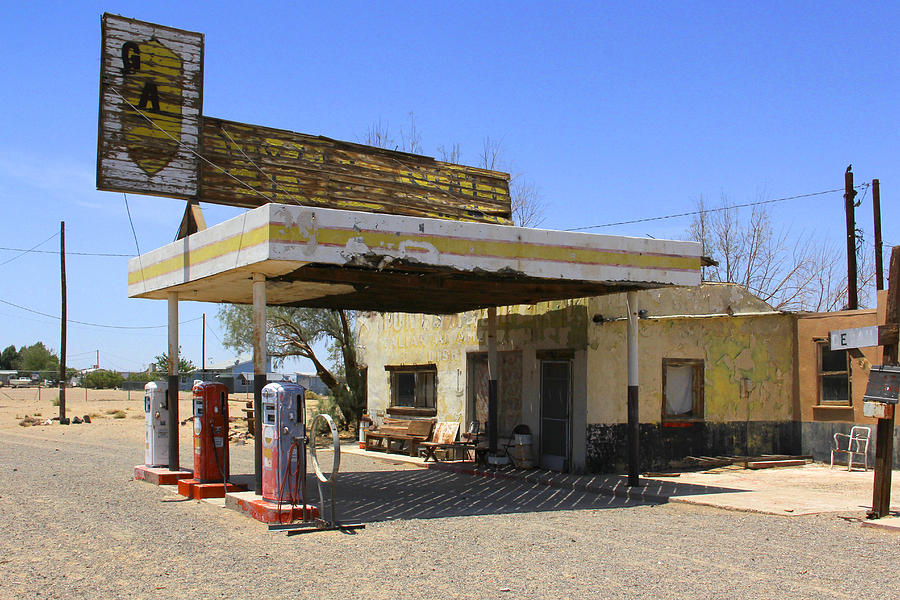The photograph captures an outdoor daytime scene of an old, abandoned gas station situated along a dusty dirt road speckled with gray gravel and yellowish sand, hinting at a desert area in the background. The gas station itself comprises a small, deteriorating adobe or stucco building with a brownish exterior and remnants of green paint that has long been chipping away. The structure features a couple of doorways and multiple intact windows, implying that it might still have some minimal use or occupancy.

Prominently visible is an overhang supported by four metal poles—rusted and exposed underneath—where three vintage gas pumps from the 1950s sit. The overhang is painted white with a yellow stripe and the exposed wood beams show signs of severe decay. The gas pumps, two red and one silver, stand beneath the rusty overhang, echoing a bygone era of roadside stops, reminiscent of Route 66.

Adding to the gas station's nostalgic feel is a weathered wooden sign above the overhang with a barely visible yellow shield logo and the letters "GA" remaining from what once spelled "GAS." To the right, an additional building with peeled yellow paint remains connected to the main structure, contributing to the eerie charm of the location. Above all this, a clear blue sky stretches overhead, completing the picturesque yet desolate image of this forsaken roadside relic.